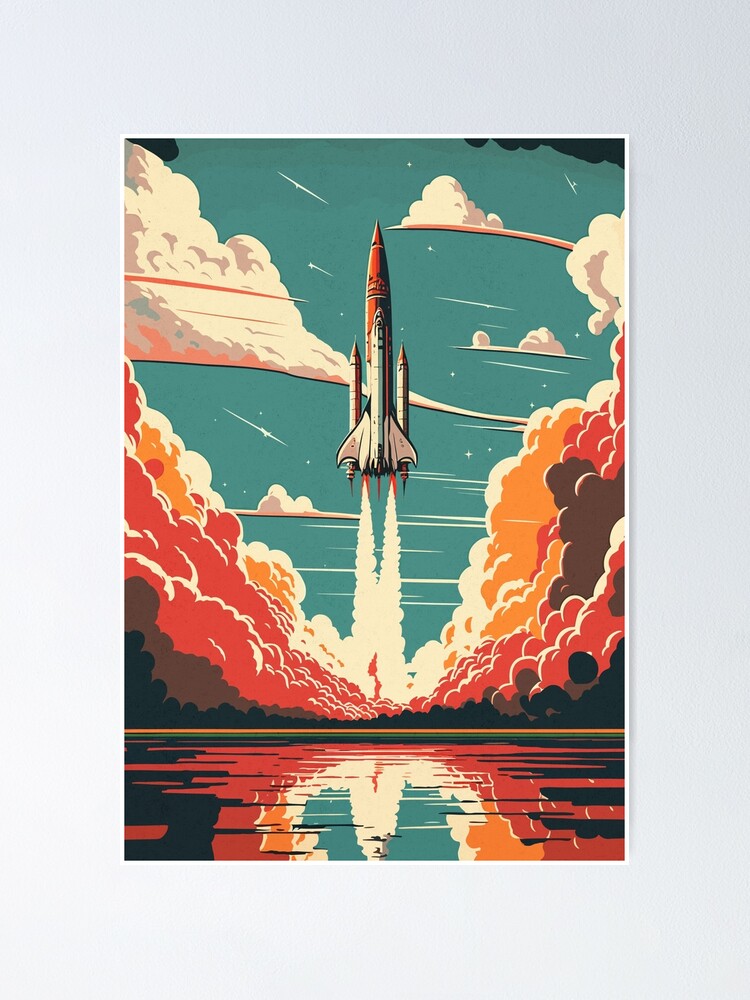This colorful illustration, reminiscent of the famous Obama painting style, depicts a robust and vibrant scene of a rocket taking off. The image is framed with a fairly thick light gray border and a slim white line, emphasizing the dynamic content within. Central to the composition, the rocket ascends into a teal, blue-green hued sky, punctuated with white clouds and faintly visible shooting star-like white strips. The rocket, characterized by its substantial size and potential to carry passengers, has a red and white exterior with three prongs and appears to have airplane-like attachments. From its base, plumes of smoke burst forth with dramatic intensity, creating a spectacular display of colors. The smoke comprises layers of red, brown, orange, black, yellow, and white, spreading outwards in vivid billows. The lower portion of the illustration shows a reflective blue-green body of water that captures the entirety of the scene above, echoing the dynamic colors and adding depth to the artwork.